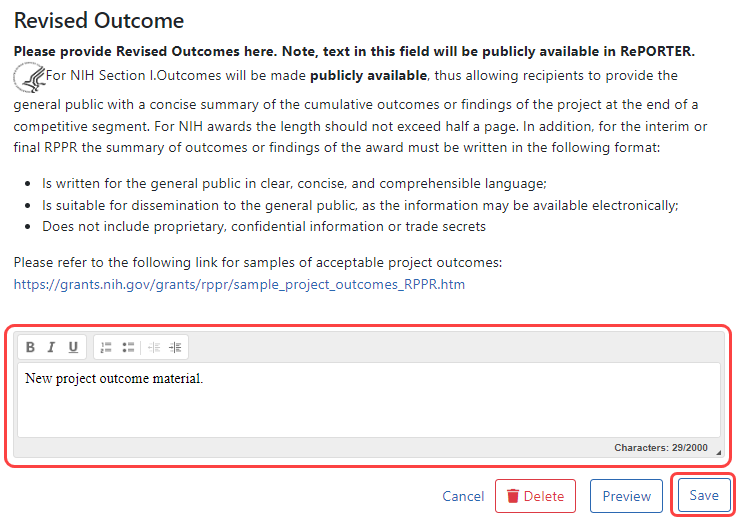Title: Instructions for Submitting NIH Project Outcomes

Caption: The screenshot displays a detailed guide for submitting project outcomes for NIH awards. At the top, bold text states, "Please provide revised outcomes here." Below, it describes the text format requirements, with a note clarifying that the text will be publicly accessible. Key points include:

- **Section 1**: emphasizes that outcomes will be made public and includes the NIH bird symbol.
- Outcomes should be summarized concisely, no longer than half a page.
- For interim or final reporting (RPPR), outcomes must be clear and accessible to the general public, avoiding proprietary, confidential, or trade-secret information.
- A linked sample is provided to illustrate successful outcome summaries.

Further instructions explain how to format text with bulleted lists, concise language, and proper indentation. At the bottom, there's a red box where users can type the new project outcome material, featuring bold, italicized, and underlined text options, along with bullet point and indent controls. It shows characters used (29 out of 22,000) and action buttons: "Cancel" in blue, "Delete" in red, "Preview" in blue, and "Save" in blue, with the "Save" button highlighted in red for emphasis.